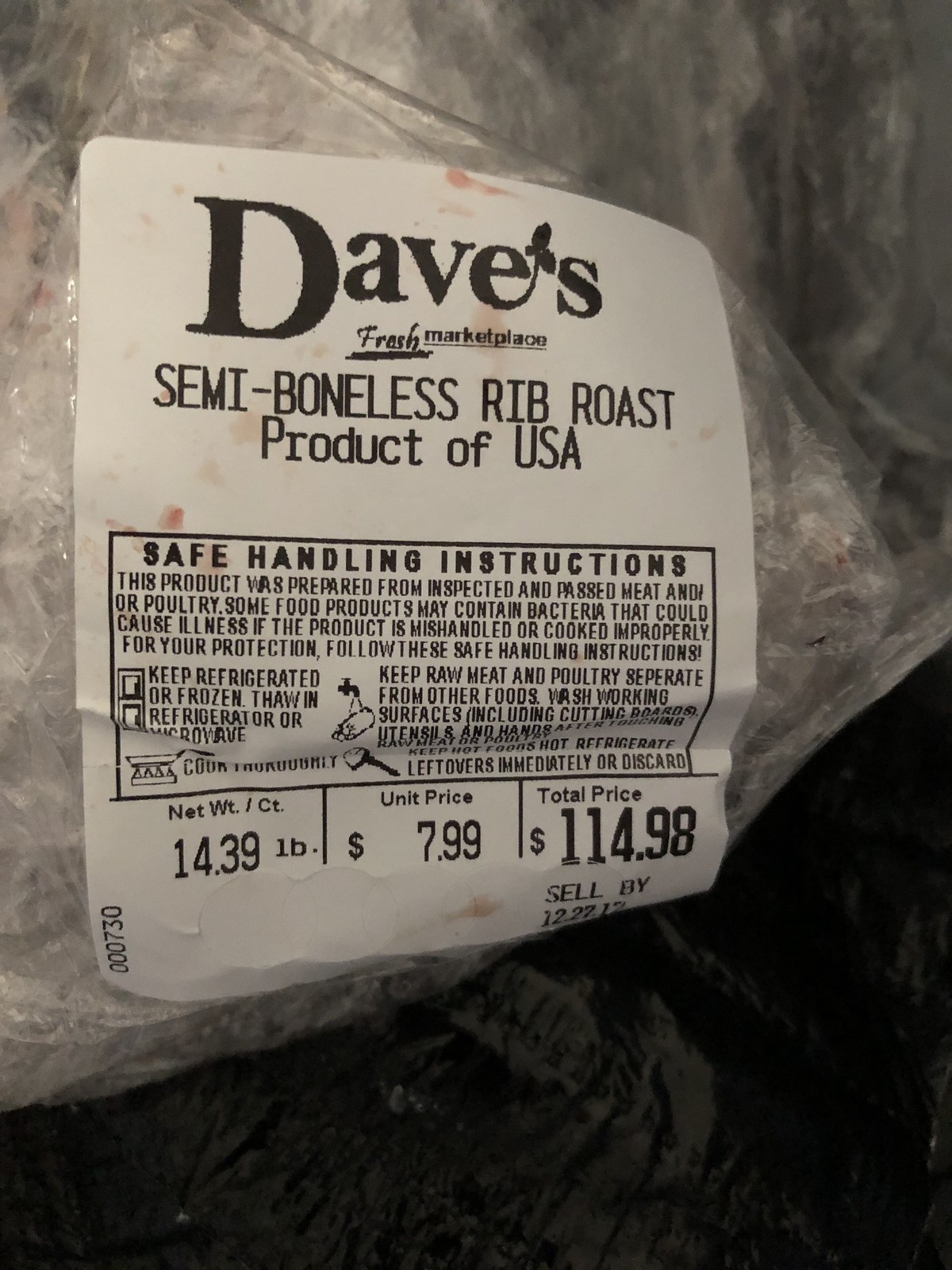This detailed indoor color close-up photograph captures a white rectangular label adhered to clear plastic packaging, likely encasing a rib roast. The majority of the background is a cellophane wrapper situated on a nearly black surface at the lower right corner of the image. The label reads "Dave's Fresh Marketplace" at the top in all lowercase letters, followed by "SEMI-BONELESS RIB ROAST" in capital letters. Below that, it specifies the product as "Product of USA." 

In the middle section, housed within a rectangle, there are safe handling instructions, including advice such as "Keep refrigerated or frozen, thaw in refrigerator or microwave." At the bottom of the label, there are details of the package: "Net Weight: 14.39 lb," "Unit Price: $7.99 per lb," and "Total Price: $114.98." The sell-by date is listed as "12-27-12." This comprehensive label provides all necessary information about the product, from its origin and handling instructions to pricing and expiration details.